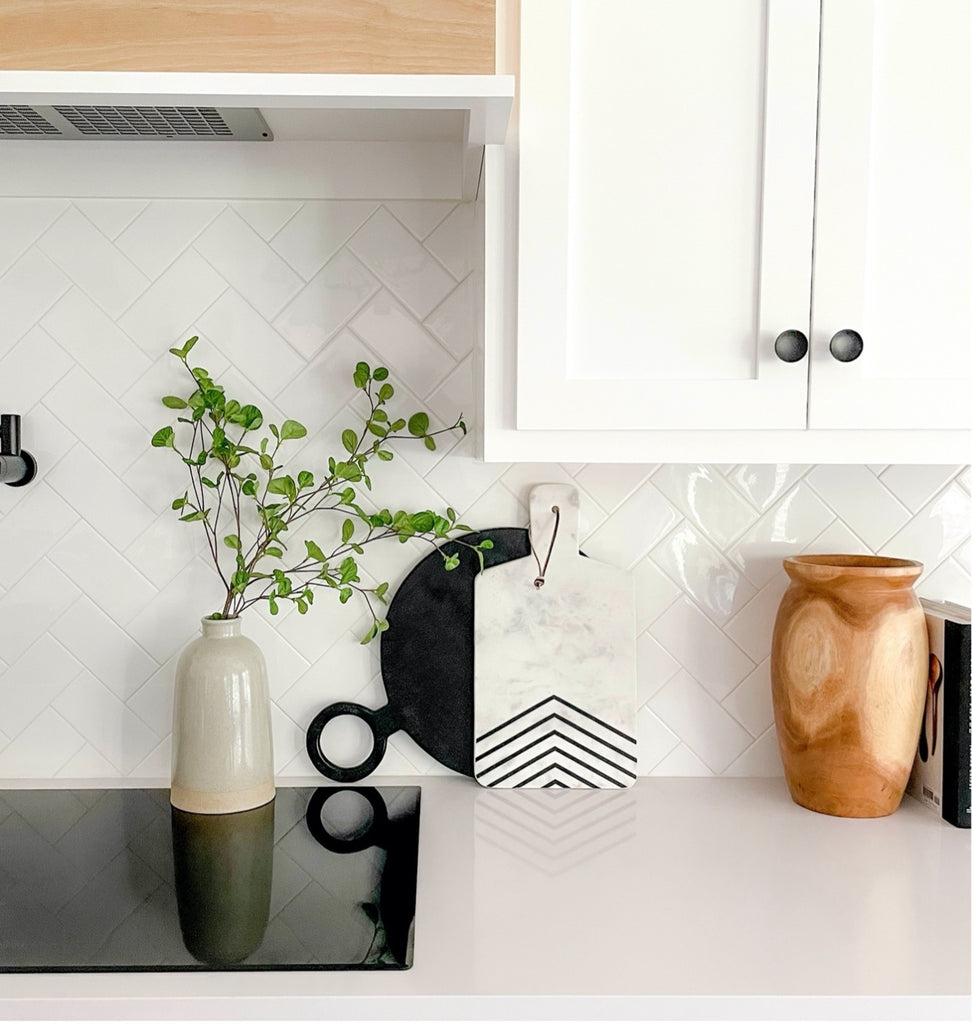The photograph depicts a modern kitchen countertop setup against a white tile backsplash. A sleek, black flat-top electronic stove occupies the center, above which there's a vent hood. In the foreground, a white countertop extends, holding a variety of carefully placed items. Dominating the scene are two vases: a tall white vase hosting several green plants or branches, and a nearby brown vase which stands empty. To the right, there's a pair of pristine white cabinets with black knobs. A white marble cutting board with subtle grey veining lies flat on the counter, accompanied by a smaller round cutting board with a unique circular handle. Additionally, a black circular board is positioned behind the cutting boards. A recipe book leans against the brown vase, adding a touch of functionality and coziness to the balanced arrangement.